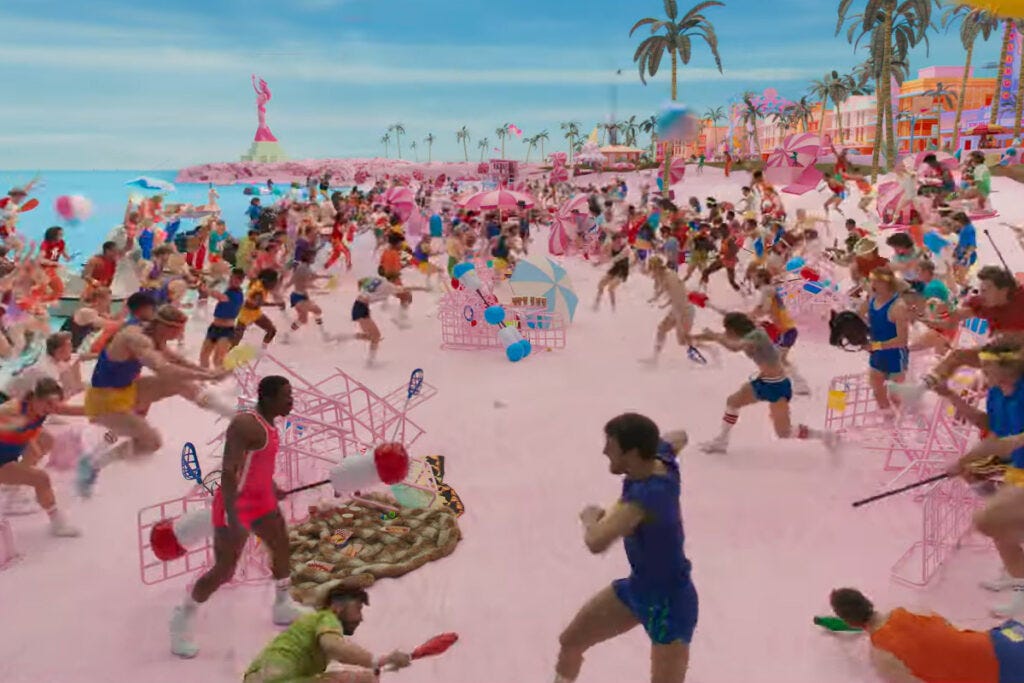The image is a vibrant, detailed still shot from the Barbie movie capturing the dramatic beach battle scene between all the Kens. They are charging towards each other from opposite sides, converging at the center of a soft pink sandy beach. The picturesque setting includes a blue sky dotted with white clouds and a striking pink Statue of Liberty in the distance. Palm trees line the shore, complementing the playful atmosphere. The beach is strewn with overturned pink lawn chairs and umbrellas, signs of the chaotic scuffle. Some Kens are sprawled on the ground, while others are emerging from the blue ocean water, each brandishing what look like oversized ear swabs as weapons. The scene exudes a colorful cacophony of motion, with bright hues of pink, aqua, yellow, and orange dominating the visual palette. Despite the lively action, no Barbies are visible in this particular shot.